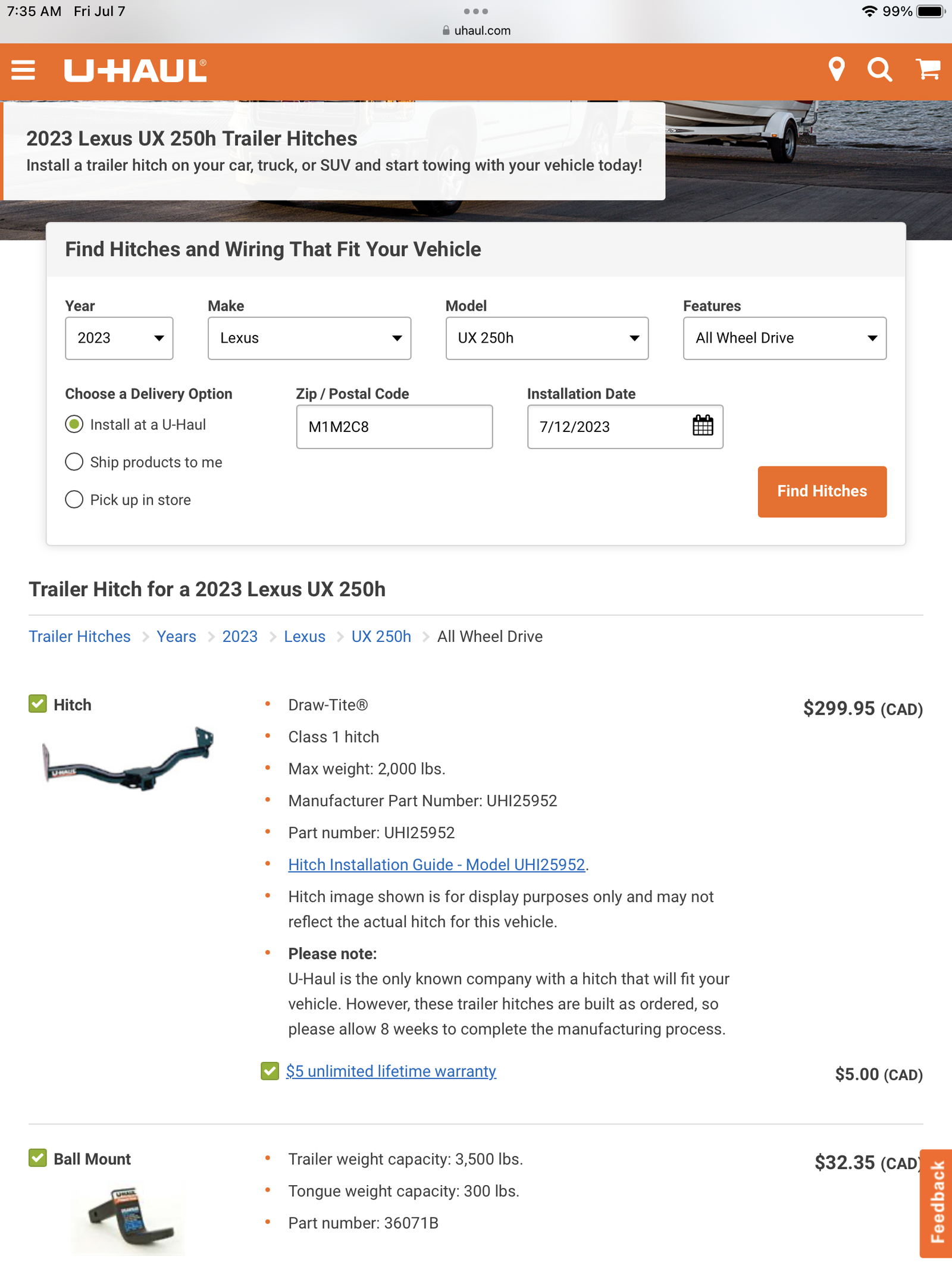The image depicts a screenshot of the U-Haul website (uhaul.com) as viewed on a smartphone or tablet. At the very top of the screen, there is a greyish-white banner displaying the device's current time (7:35 AM), date (Friday, July 7th), and battery life (99%). Directly below this is an orange navigation bar featuring the U-Haul logo on the left and icons for search and shopping cart on the right.

Below the navigation bar, a promotional banner shows an image of a boat trailer, with a white overlay panel displaying the text "2023 Lexus UX 250H Trailer Hitches." 

Further down, a search form allows users to enter the year, make, model, and features of their vehicle. This section includes options for delivery, a field to enter a zip code, an installation date selector, and an orange "Find Hitches" button located in the bottom right corner of the form.

At the bottom of the screenshot, search results are displayed. The first result features a trailer hitch priced at $299.95 CAD, with its product details listed on the right. The second result showcases a ball mount priced at $32.35 CAD, also accompanied by product details on the right.